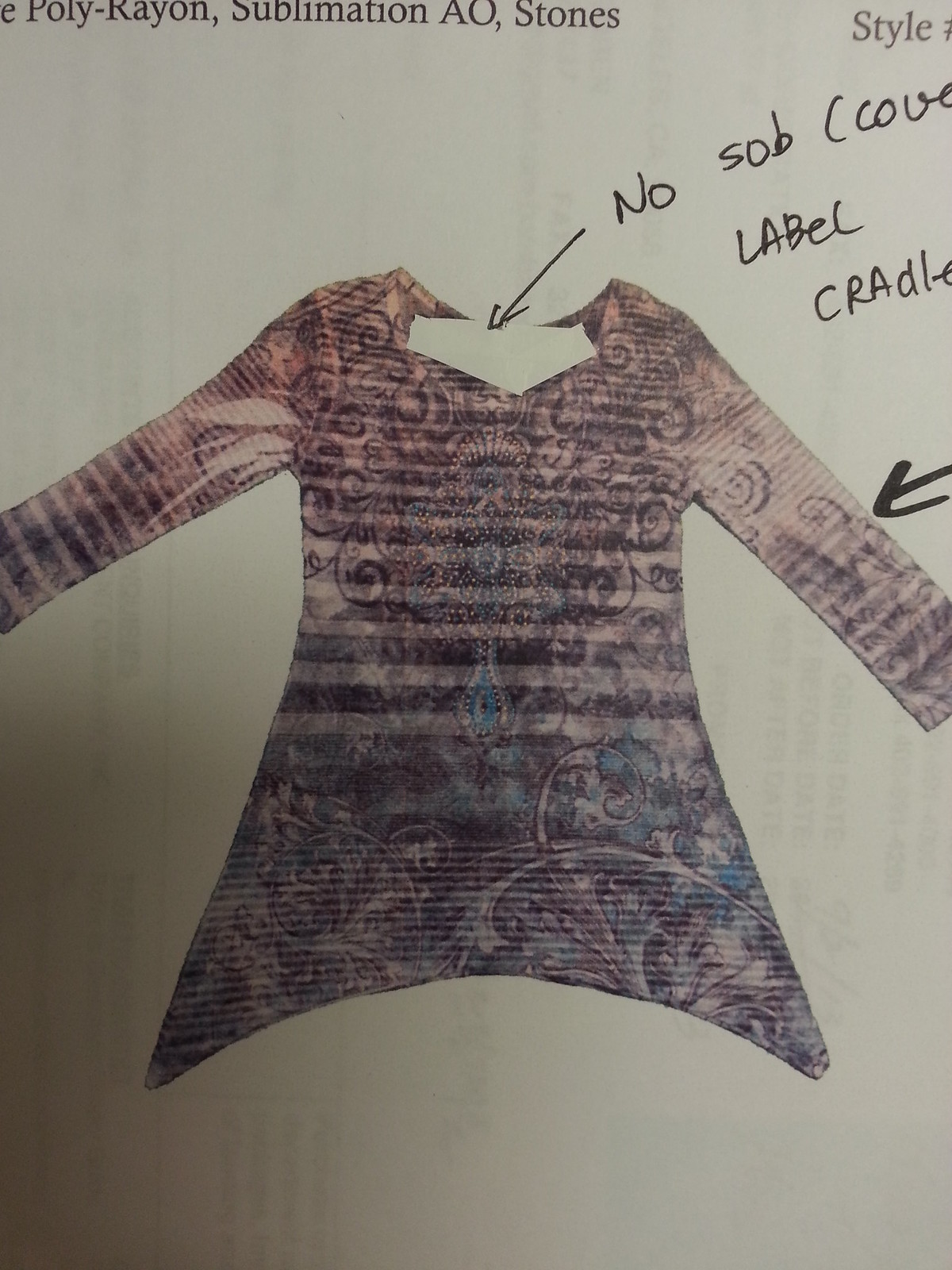The image depicts a piece of paper with a detailed drawing of a long-sleeved shirt. The shirt, which appears to be a grayish or white garment, features a distinct purple flowery pattern, including a central floral vase design with sparkly stars and grass vine motifs near the bottom sides. At the top left of the paper, there is typewritten text stating "Poly Rayon Sublimation AO, stones." In addition, there are handwritten annotations in black ink: one arrow points to the neckline, accompanied by the words "no SOB cover label cradle," and another arrow pointing towards the right sleeve, although the sleeve and its label are partially out of frame. The top right corner of the image includes the handwritten word "style."